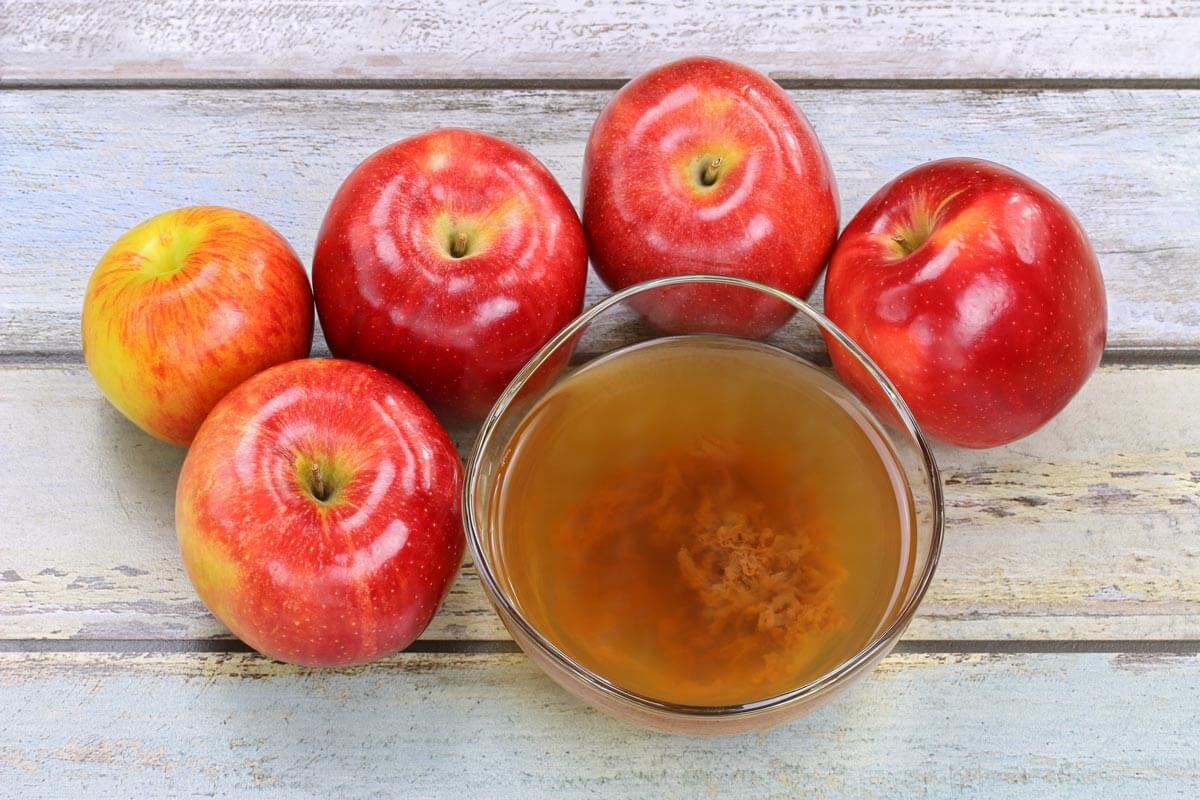An overhead view captures five ripe red apples of varying shades, from dark red to light yellow-green, arranged on a distressed white wooden slatted table. Each apple, with its short, shiny stem, is positioned so their tops are visible. The apples stand upright, though some are slightly angled. Nestled among them is a clear glass bowl filled with freshly blended apple cider, characterized by its yellowish-brown hue and suspended, chunky apple bits. The rustic tabletop, with its visible brown scratches and streaks, enhances the scene's vintage charm.